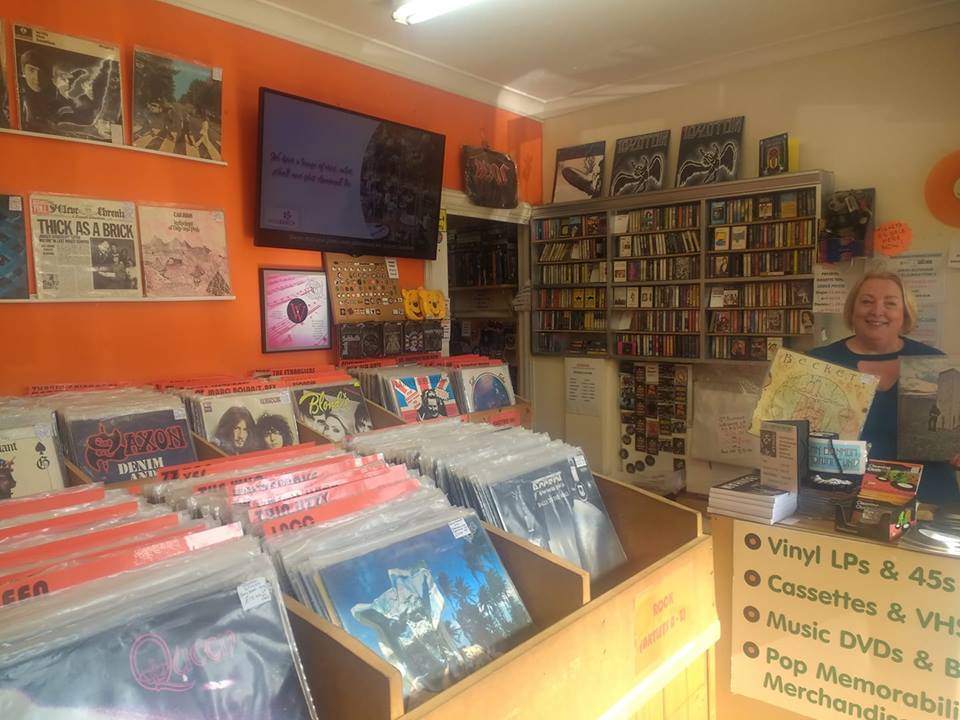The indoor photograph depicts a small vintage-style vinyl record store with vibrant colors and nostalgic decor. On the left side, a display shelf holds a collection of vinyl albums encased in plastic sleeves. Behind this shelf, the back wall is painted a vivid orange and adorned with iconic vintage records, including those of The Beatles and Led Zeppelin, as well as newspaper articles. A large flat-screen TV is mounted on the wall above. On the right side of the image, a younger, somewhat heavyset blonde woman stands behind a counter, smiling and holding up an album. The counter features a sign with green lettering that lists the store’s offerings: vinyl LPs and 45s, cassettes and VHS, music DVDs, pop memorabilia, and merchandise. Further behind her is a rack filled with CDs and cassette tapes. The overall ambiance is cozy and nostalgic, inviting customers to browse through a diverse collection of music and memorabilia.